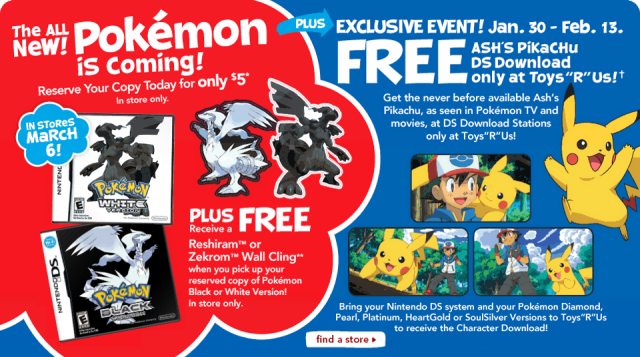**Detailed Caption:**

This advertisement enthusiastically promotes the release of new Pokémon games, featuring vibrant and eye-catching elements. On the left side of the ad, within a bold red, cloud-shaped design, a prominent message announces: *"The all-new Pokémon is coming. Reserve your copy today for only $5, in-store only. Available March 6th!"* Beneath this announcement, two game covers are displayed – *Pokémon Black* and *Pokémon White*. Each cover showcases iconic characters from the games, creating a sense of excitement and nostalgia.

Additionally, the advertisement highlights a special offer: *"Plus receive a free Reshiram or Zekrom Wild Cling when you pick up your reserved copy of Pokémon Black or White version. In-store only."*

On the right side of the ad, there’s another exclusive event promotion running from *January 30th to February 13th*. It details a unique opportunity to obtain *Ash's Pikachu* via a DS download at *Toys "R" Us* locations. A description reads: *"Get the never-before-available Ash's Pikachu as seen in Pokémon TV and movies at DS download stations only at Toys 'R' Us."* Above this description, there are three screen captures from the anime featuring Ash and Pikachu, while an image of Pikachu mid-jump adds dynamic energy to the visual.

At the bottom of the ad, a white text segment on a contrasting background advises: *"Bring your Nintendo DS system and your Pokémon Diamond, Pearl, Platinum, HeartGold, or SoulSilver versions to Toys 'R' Us to receive the character download."* 

Finally, a white button with red lettering saying *"Find a Store"* is positioned at the bottom left of the ad, guiding customers to locate their nearest retailer. The overall ad captures the excitement and urgency of these Pokémon releases and special events, appealing to fans and collectors alike.